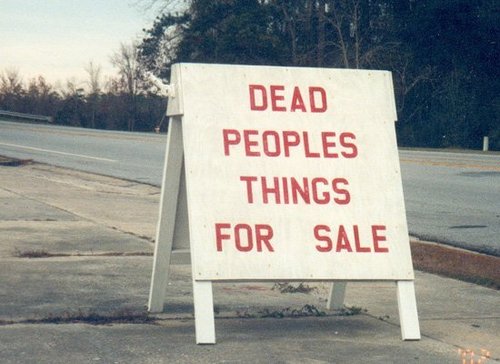This photograph captures a somewhat eerie scene along a single carriageway road flanked by a dense forest of trees and bushes. The sky is slightly faded, perhaps hinting at an older or edited image. Dominating the foreground is a large, white wooden placard sign shaped like a triangle, somewhat resembling a sawhorse, and stenciled in stark, red capital letters with the unsettling message: "DEAD PEOPLE'S THINGS FOR SALE." Interestingly, the word "PEOPLE'S" lacks an apostrophe, leaving its intention ambiguous. The sign is settled on massive paving slabs with weeds peeking through the cracks, adding an element of neglect. Further down, a grey crash barrier suggests an upcoming bend in the road. The road itself is faded and devoid of vehicles, lending a deserted, almost haunting atmosphere to the scene, accentuated by the surrounding forest and the absence of any residential structures.